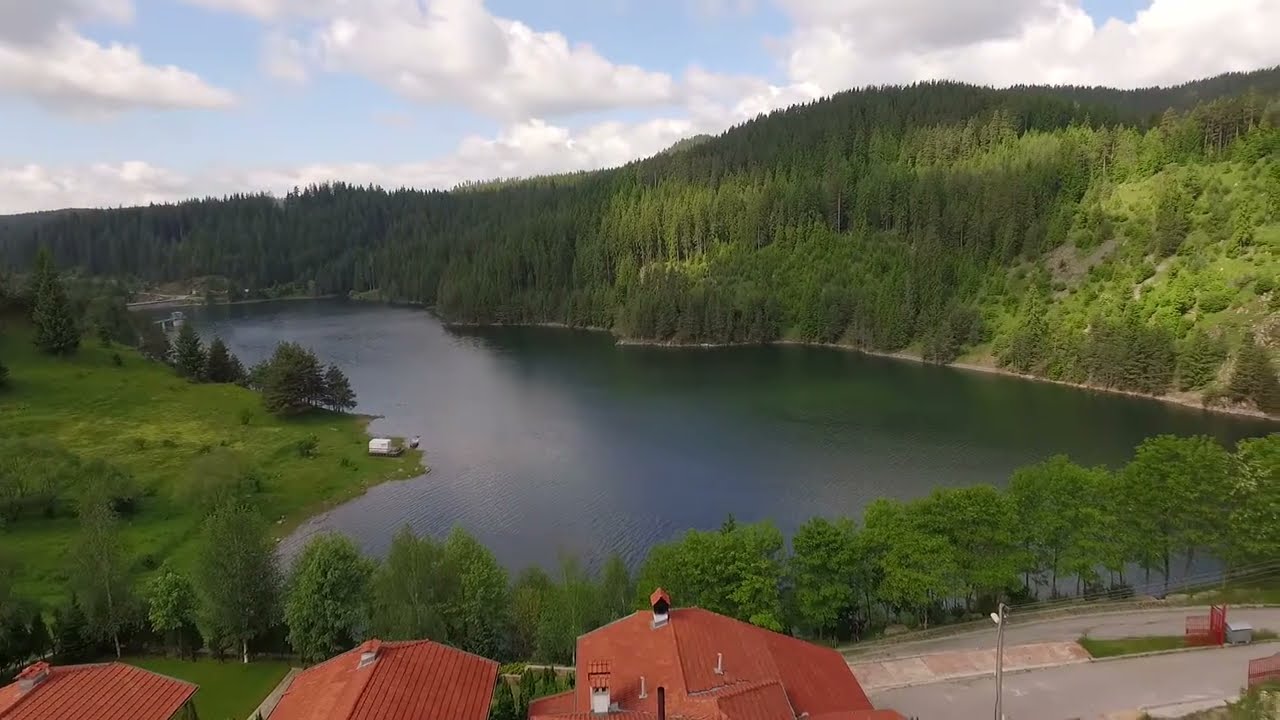This elevated, high-angle shot captures a tranquil, picturesque lake nestled in a lush, mountainous setting. The scene appears to be taken from a drone or tall vantage point, providing a sweeping view of the natural beauty. The lake, of moderate size, is surrounded by varied landscapes: to the right, a densely forested hillside teeming with evergreen trees slopes gently down to the water; to the left, the shoreline opens up into a sprawling grassy area, where a truck and trailer are parked, with a canoe or small boat visible on the lake. 

In the foreground, three buildings with striking red rooftops punctuate the green expanse, possibly lodges or residences, situated next to a paved parking lot and a road that winds along the edge of the lake. There is a sign near the parking area, hinting that one of these structures might be a restaurant or similar facility. Additionally, a small white house can be observed on the left shore. The sky above is a brilliant blue, adorned with fluffy white clouds, making the overall scene look cozy and inviting. Down by the lake, a lone figure appears to be fishing, adding a touch of human presence to this serene landscape.